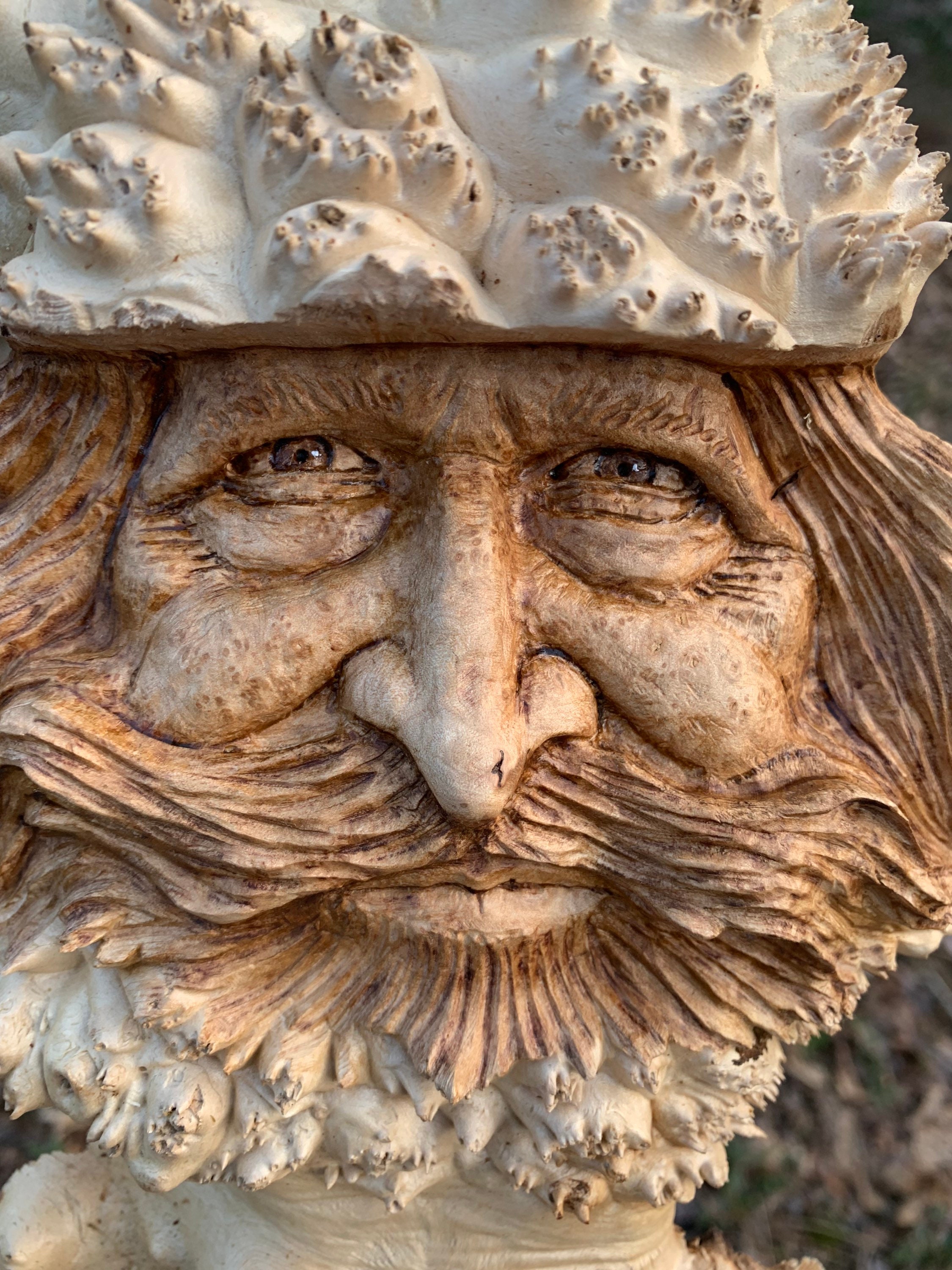The photograph showcases a meticulously crafted wood carving, possibly made from maple-burled wood, depicting the face of an older man. The man is adorned with a long, brown mustache and a well-defined beard. His longer hair extends to the sides of his head, adding to his rough and weathered appearance. The carving is polished to reveal intricate details, including piercing, realistic-looking brown eyes and a sharp nose. The man wears a crown or hat with a rough texture, whiter in color, resembling seashell-like points or waves. His coppery, orange-brown face, possibly weathered by the elements, exudes warmth and a sense of ancient wisdom. Wrinkles around his kind eyes and a subtle smile suggest a life filled with stories. The grey background contrasts with the lively tones of the carving, emphasizing the intricate craftsmanship of this detailed wood art.